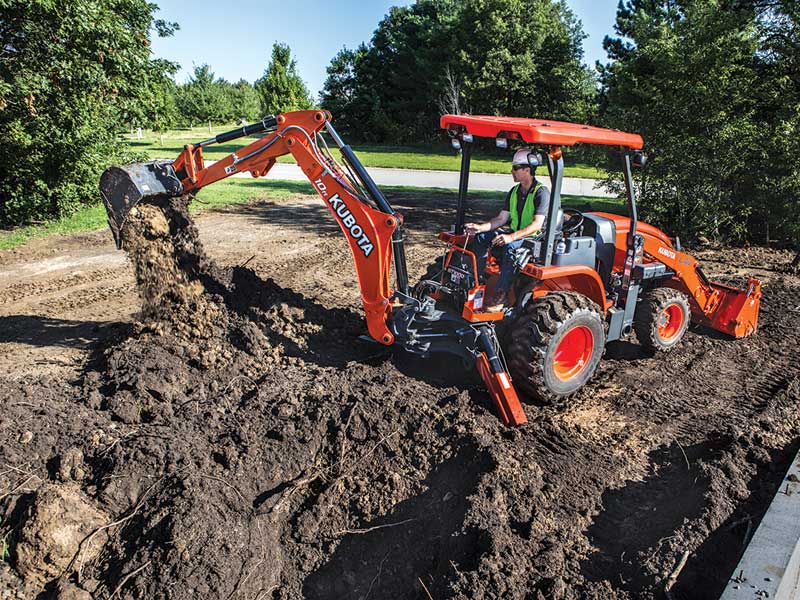This detailed outdoor photograph captures an action shot of a man operating an orange Kubota excavator. The machine, which features large black wheels, is actively scooping and pouring dirt onto a patch of uncovered dark brown soil. The operator, dressed in jeans, a black t-shirt with a yellow reflective safety vest, and a white construction helmet, is holding the controls with a focused demeanor. He is also wearing black sunglasses to shield his eyes from the bright daylight. The scene is set against a backdrop of lush green trees and a light gray road or wide walking path, indicating the location might be a park. The atmosphere suggests a warm, sunny day, with a clear blue sky overhead. The soil being moved by the excavator seems to contain roots, highlighting the machine’s engagement with the natural terrain.